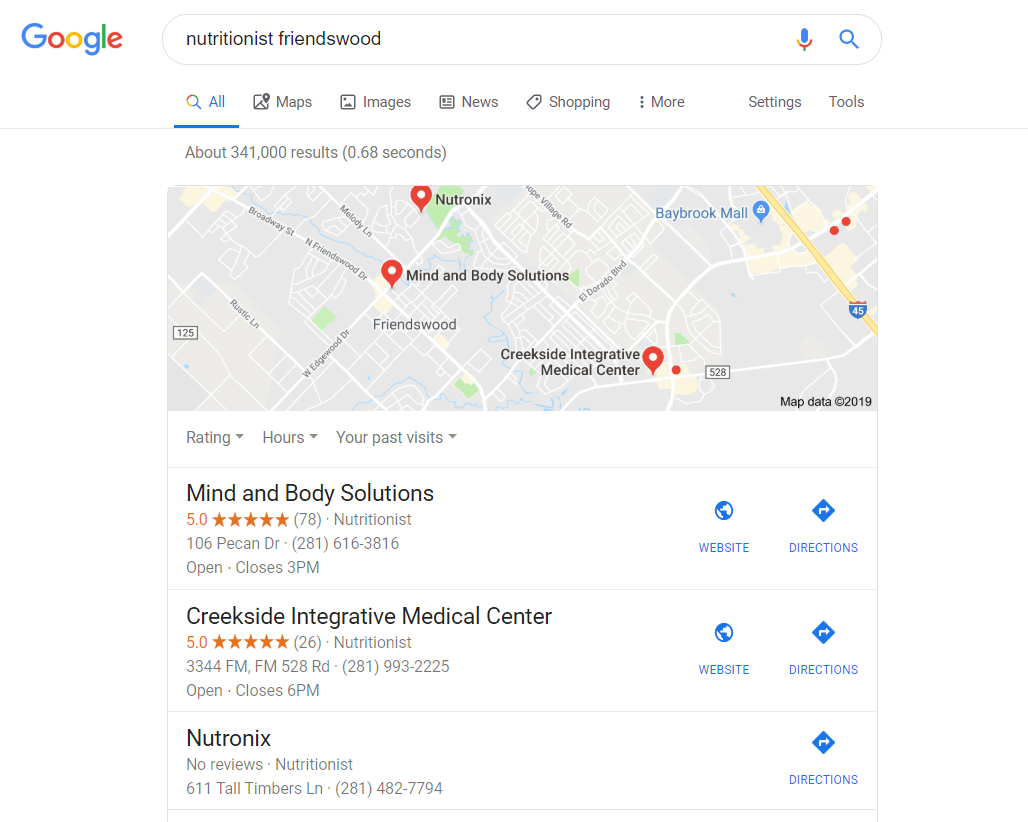The image is a screenshot from a Google search, possibly taken from a tablet or a desktop. The interface has a white background at the top, prominently displaying the Google logo with its multicolored letters—blue 'G', red 'o', yellow 'o', blue 'g', green 'l', and red 'e'. To the right of the logo is an elongated search box spanning the width of the screen, where the search term "nutritionist friends would" has been entered.

Directly below the search box are various tabs for refining search results, such as "All," "Maps," "Images," "News," "Shopping," and "More." The "All" tab is selected. The first result displayed is a Google Maps snippet showing a top-down map of the Friendswood area, marked with red pins indicating medical facilities. Three notable locations are highlighted: Mind and Body Solutions, Creekside Integrated Medical Center, and Neutronics. Below the map, details for these businesses are listed, including their names, star ratings, addresses, and contact information.